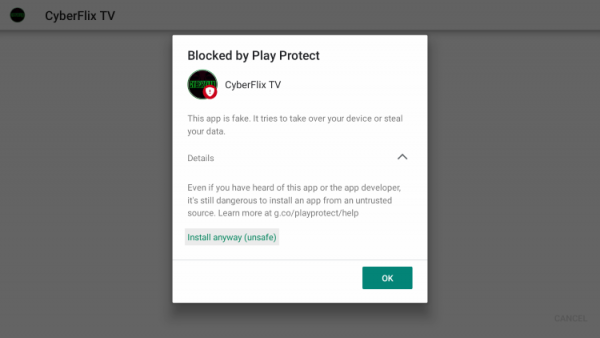The image appears to be a screenshot from a website interface displaying a pop-up warning from Google Play Protect. The background of the image is light gray with a hazy, cloudy appearance, indicative of the standard overlay used when a modal or pop-up is displayed. 

In the top left corner of the background, there is a black circle, next to which "CyberFlix TV" is written in bold black letters. "CyberFlix" is in one word followed by "TV" in capital letters.

The central focus of the image is the pop-up tab, which occupies a substantial portion of the screen, approximately one inch from the top and bottom edges, and three inches from the left and right edges. The background of the pop-up is white.

At the top of the pop-up, in bold black text, are the words "Blocked by Play Protect". Below this, there is a black circle featuring green lettering that is indistinct. In the bottom left portion of this black circle, there is a smaller red circle containing a white shield with a red exclamation point inside it. To the right, it reads "CyberFlix TV".

Following this, the warning message states: "The app is fake. It tries to take over your device or steal your data." Then, it prompts the user towards more information with a link labeled "Details" followed by an arrow pointing up.

Further down, the warning continues: "Even if you have heard of this app or the app developer, it's still dangerous to install an app from an untrusted source." It then provides a link for more information: "Learn more at g.co/PlayProtect/help".

At the bottom of the tab, there is a gray button with green text reading "Install Anyway" and a cautionary note in quotations, "unsafe", separated by a thin gray line. In the bottom right corner of the pop-up, there is a green button labeled "OK" and another option, "Why".